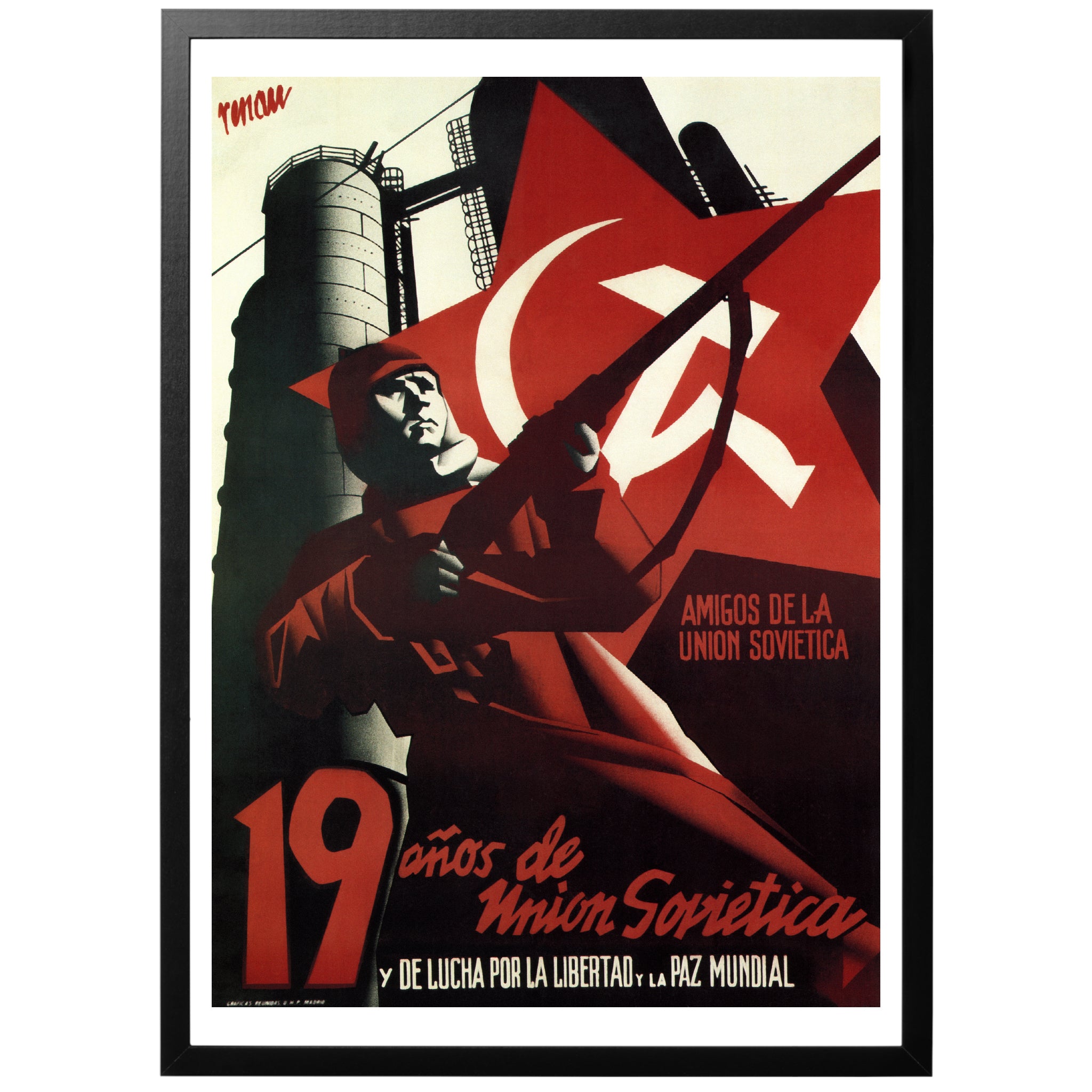The image is of a detailed war propaganda poster, prominently showcasing Soviet Union themes. Central to the poster is a man dressed in a red uniform, holding a long-barreled rifle with a noticeable strap. The background features industrial elements such as power plants, ladders, a bridge, and a watchtower, symbolizing a stark industrial environment often associated with Soviet imagery. A large red star and Soviet symbols, including a white half-circle with a hammer, are present, enhancing the propagandistic feel. Text in the image, not in English, reads "Amigos de la Unión Soviética, 19 años de la unión soviética y de lucha por la libertad y la paz mundial," emphasizing the poster’s message of solidarity with the Soviet Union and its fight for freedom and global peace. The poster is framed with multiple layers, including a white and a black frame, further reinforcing its presentation as a significant and carefully crafted piece of propaganda.